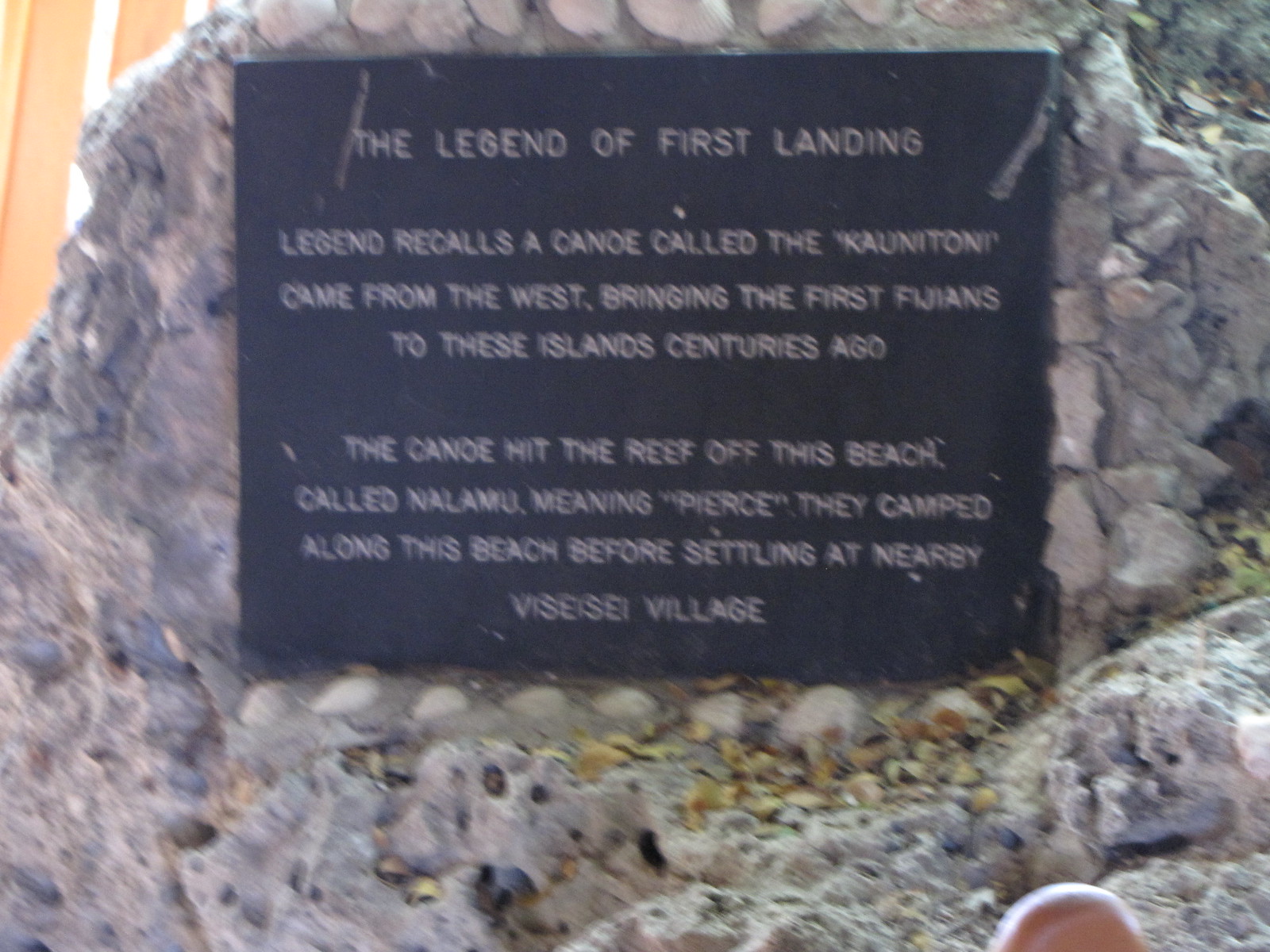This image captures a somewhat blurry photograph of a memorial plaque mounted on a large, bumpy gray rock formation. The plaque, which is black and hung vertically, features white or light gray text that reads, "The Legend of First Landing." The text details the historic legend of a canoe called the Kaunitoni that arrived from the West, bringing the first Fijians to these islands centuries ago. According to the legend, the canoe hit the reef off a beach called Nalamu, which means "pierce." The first Fijians camped along this beach before eventually settling in the nearby Visesei village. In the background, natural light illuminates the scene, and in the top left corner, a peach-colored blur is visible. Additionally, a small portion of a finger appears at the edge of the photo, indicating it may have been inadvertently captured by the person taking the picture. Small rocks and pebbles litter the ground around the large rock, adding to the rugged natural setting.